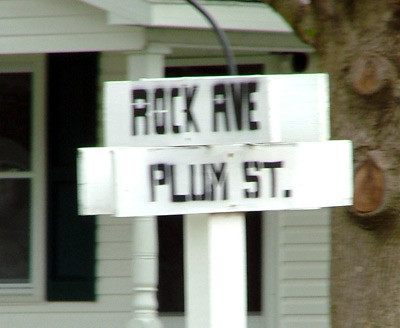This image showcases a somewhat blurry photograph of a street corner, dominated by a white street signpost made of wood. Affixed to the post are two small rectangular signs: the top one reads "Rock Avenue" in black text, while the bottom one displays "Plum ST" with a period. The signs are designed to be readable from both directions. To the right of the street sign, a large tree trunk with visible brown bark and two circular knobs where branches have been cut off extends vertically through the image. In the background, partially visible, is a white house with black shutters and white siding. The house's roof, also white, can be seen in the composition.